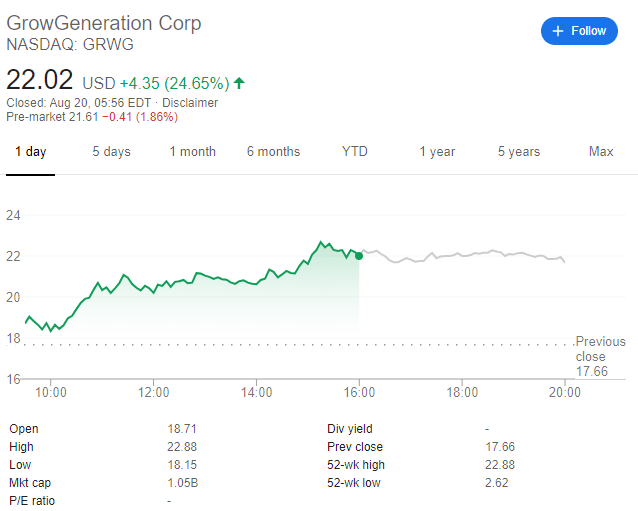This image features a detailed snapshot of a stock performance graph for GrowGeneration Corp, traded on NASDAQ under the ticker symbol GRWG. In the top right corner, an option to "Follow" the stock is available. Prominently displayed in large numbers, the stock price is $22.02 USD, reflecting an increase of $4.35, or 24.65%, indicated by an upward green arrow. The market closed on August 20th at 05:56 EDT, as noted on the image, followed by a disclaimer. Below this, pre-market information shows a price of $21.61, a decrease of $0.41 or 1.86%. The bottom part of the image includes a graph with options to view data over various time frames: 1 day, 5 days, 1 month, 6 months, year-to-date (YTD), 1 year, 5 years, and max. The graph depicts a generally upward trend with some intermittent declines, illustrating overall growth. The graph is annotated with axes and sections to breakdown the data points, providing a comprehensive visualization of the stock's performance trends.